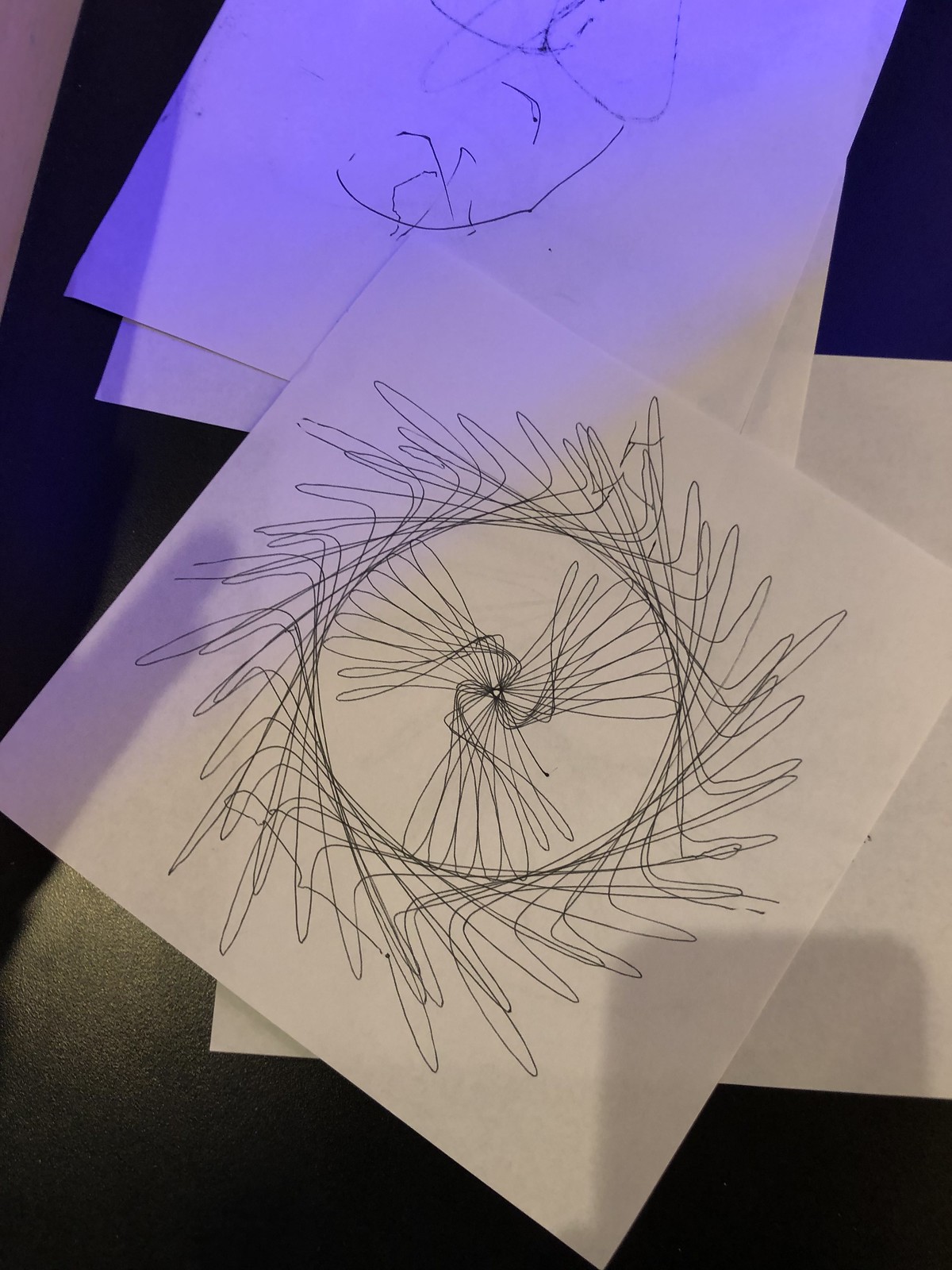On a stark black background, four sheets of square paper lay scattered with a seemingly random arrangement. In the upper left corner of the image, a small area of darker gray interrupts the black, while on the bottom left, a patch of tan color breaks through the darkness. The bottom right corner features a partial square shadow in a medium gray tone.

The focal point of the image is a sheet of white paper, placed slightly rotated to create a diamond shape. In the center of this paper, there is a hand-drawn circle, likely created using a drawing compass or an object as a stencil. Surrounding the circle is a series of uniform scribbles, drawn with a black pen. These scribbles attempt to form a consistent pattern, reminiscent of designs made with a spirograph drawing toy. However, the inconsistencies and occasional errors around the exterior and interior of the circle reveal the human touch in its creation, giving the piece a unique, imperfect charm.